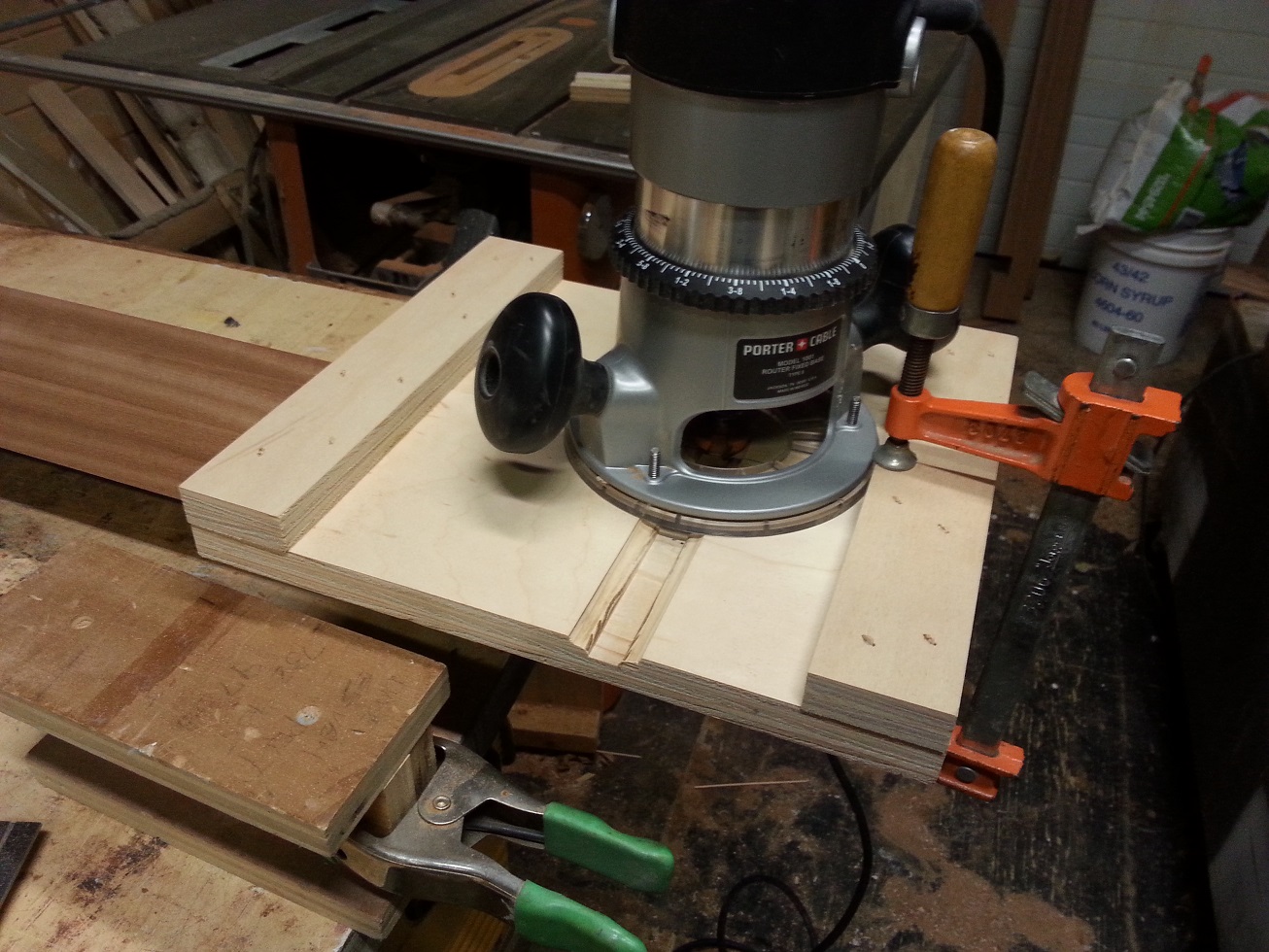The image showcases a bustling woodworking shop, centered on an intricate setup for a woodworking project. At the heart of the image is a Porter Cable router, identifiable by its cylindrical shape and branding, with a black top that transitions into gray, and a metallic lower section. This router is actively cutting into a light wooden piece, which features an indented groove, held securely in place by an orange clamp with a wooden handle on the left. Adjacent to this, at a lower elevation, another piece of wood is secured by a green clamp, suggesting a layered or glued assembly.

To the left side of the image, various wood planks and additional tools are visible, emphasizing the clutter and activity typical of such workspaces. In the background, a metal bench can be seen, adding to the utility and storage space in the shop. On the far right, a white bucket topped with a bag, presumably of corn syrup, and scattered wood pieces denote the room's utilitarian use. Above this bucket, sections of a white plaster wall and bricks provide a subdued backdrop to the scene. The workspace floor is littered with sawdust, reflecting recent activity and the ongoing nature of projects within this detailed and industrious environment.